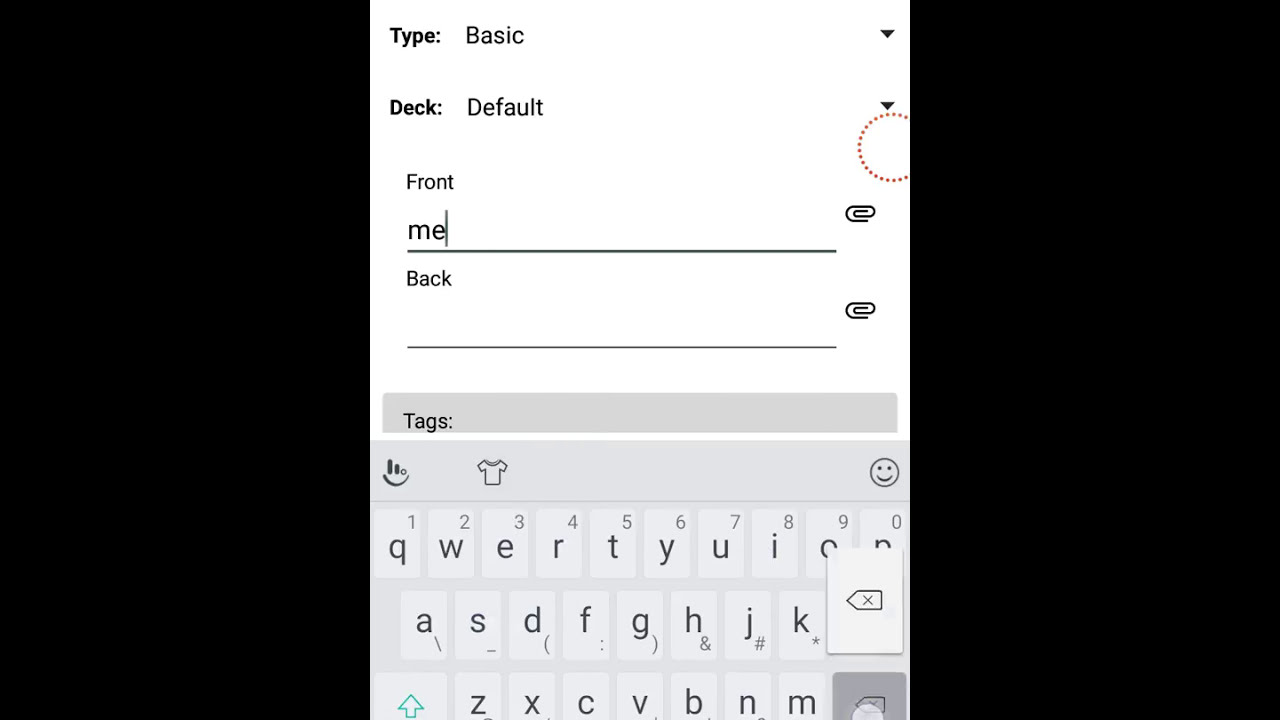This is a screenshot depicting a white keyboard layout against a white background, formatted in a vertical orientation. Central to the image is a horizontal black bar, featuring white text that reads: "Type: Basic (deck: Default)". Below this, the segment marked "Front" displays the word "me" partially typed, indicated by a cursor line, suggesting that typing is in progress. The section labeled "Back" underneath this remains blank.

Flanking the right-hand side of the screen, there are a series of interface elements: starting from the top, a return arrow, followed by two drop-down arrows, a dotted circle facing right, and two paper clip icons, indicative of attachment features. The word "tags" is positioned below these elements.

The keyboard shown at the bottom is a standard QWERTY layout. The visible portions include the keys: QWERTYUI on the top row (with the last two letters obscured), the complete set of ASDFGHJK keys in the middle row, and the ZXCVBNM keys in the bottom row, fully displayed.